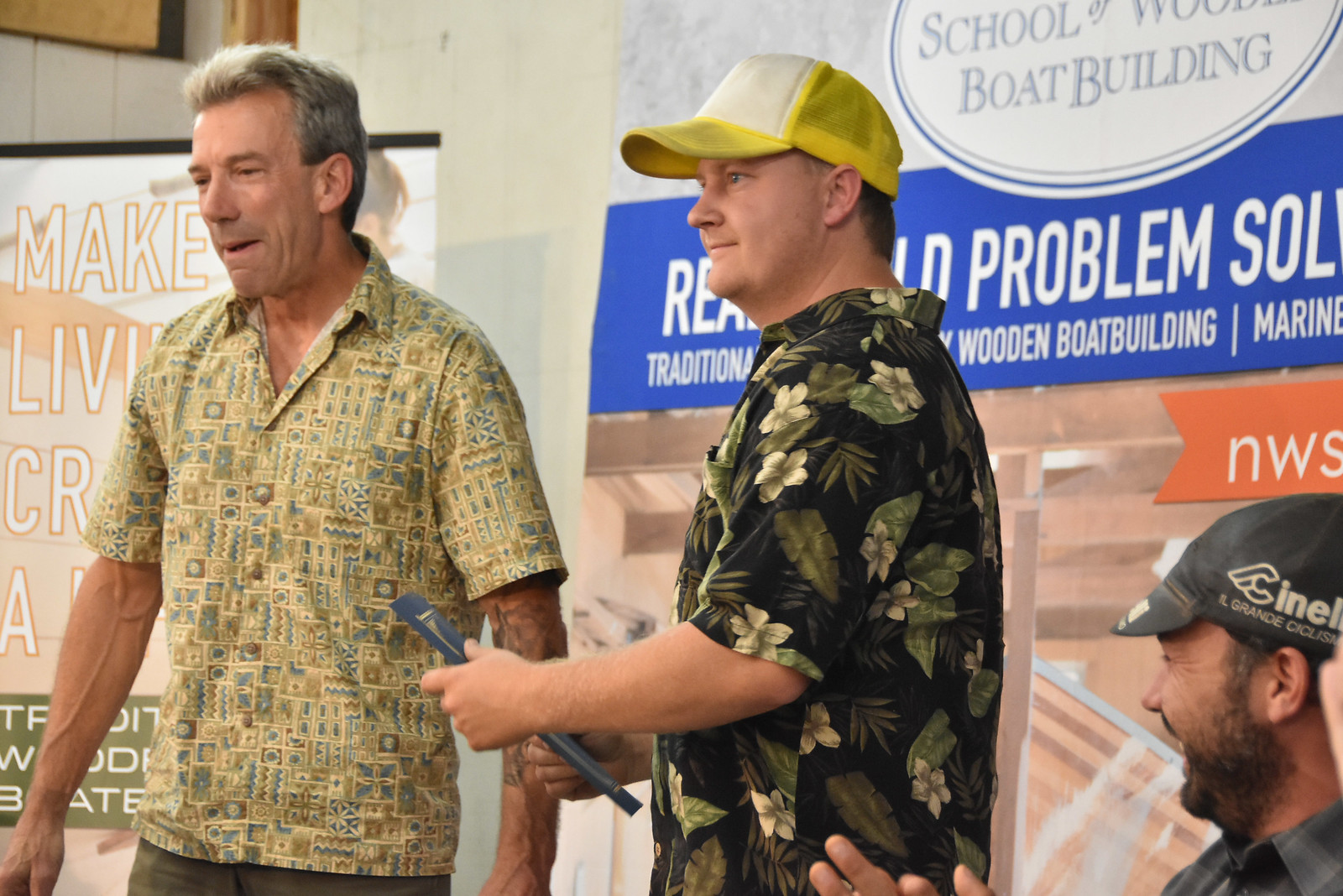In the image, three men appear to be on an elevated podium or stage, participating in a celebration or award ceremony at the "School of Wooden Boat Building." The man on the left is wearing a short-sleeved button-up shirt that reaches just above his elbows. The man in the middle stands out with his floral Hawaiian shirt and a distinctive white and yellow mesh trucker’s cap. He is holding a piece of paper or cardboard, which adds to the impression that they are presenting or receiving an award. On the right, a bearded gentleman is smiling and clapping, wearing a black baseball hat. Although much of the background text is obscured, the visible words include phrases like "school," "boat building," "problem solving," "marine tradition," and "traditional wooden boat building." All three men exude happiness, underscoring the celebratory nature of the event.